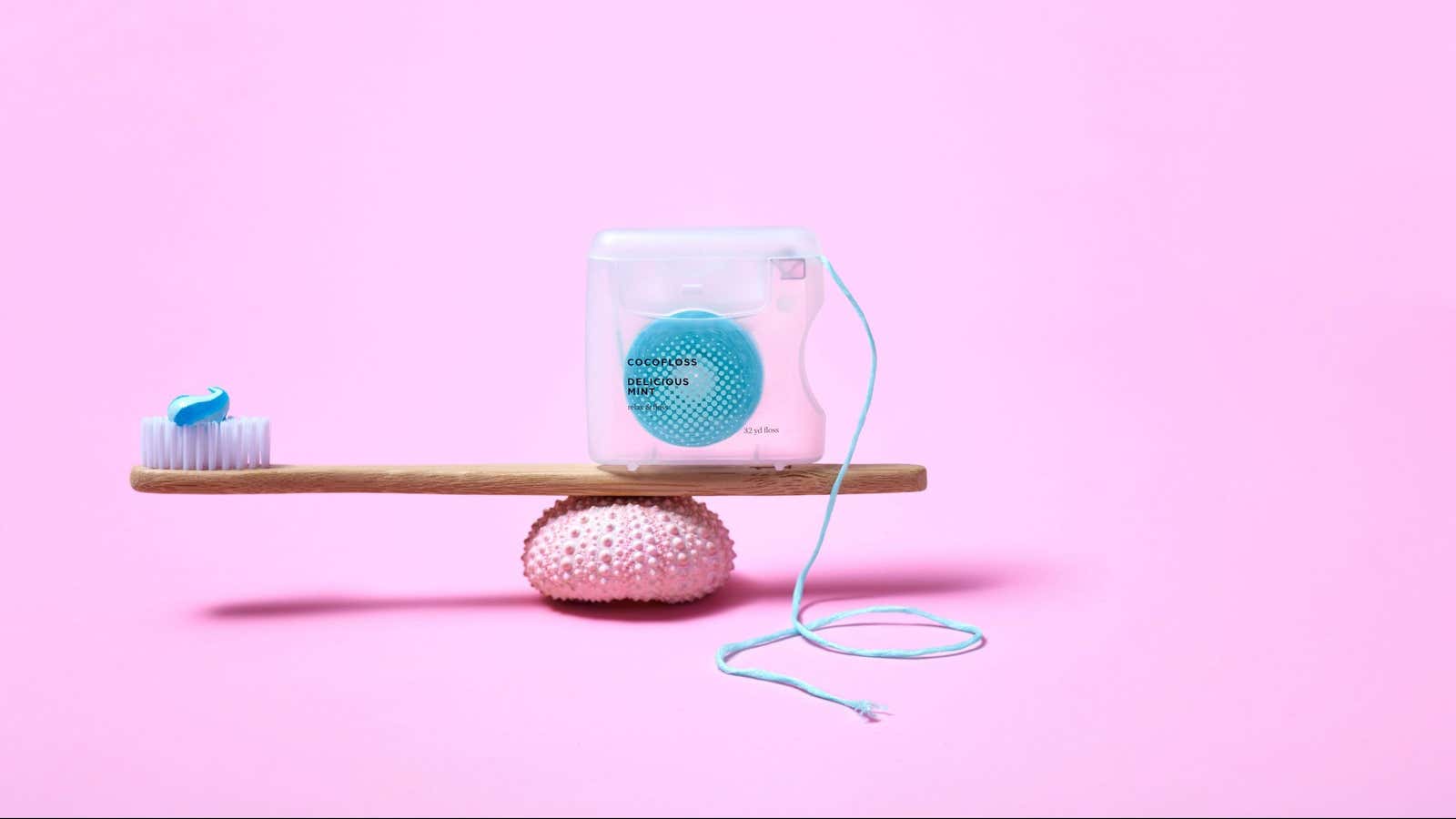In this photograph with a vibrant bubblegum pink background, an array of objects is artfully arranged. At the bottom of the image lies a light pink, textured, oval object resembling a flattened, spiky ball or cushion. Resting atop this object is a wooden toothbrush with white bristles, casting a distinct shadow onto the surface below. The toothbrush is oriented with its bristles pointing to the left side of the image. On the bristles, there is a swirl of dark blue toothpaste with a white stripe in the middle. Positioned towards the bottom end of the toothbrush handle is a clear plastic dispenser labeled "Coco Floss," though the black text is partially unreadable. The translucent dispenser reveals a spool of teal or cyan-colored dental floss, some of which is unwound and dangles in a loop onto the pink surface. The detailed placement and textures of these items create an intriguing visual display against the vivid background.